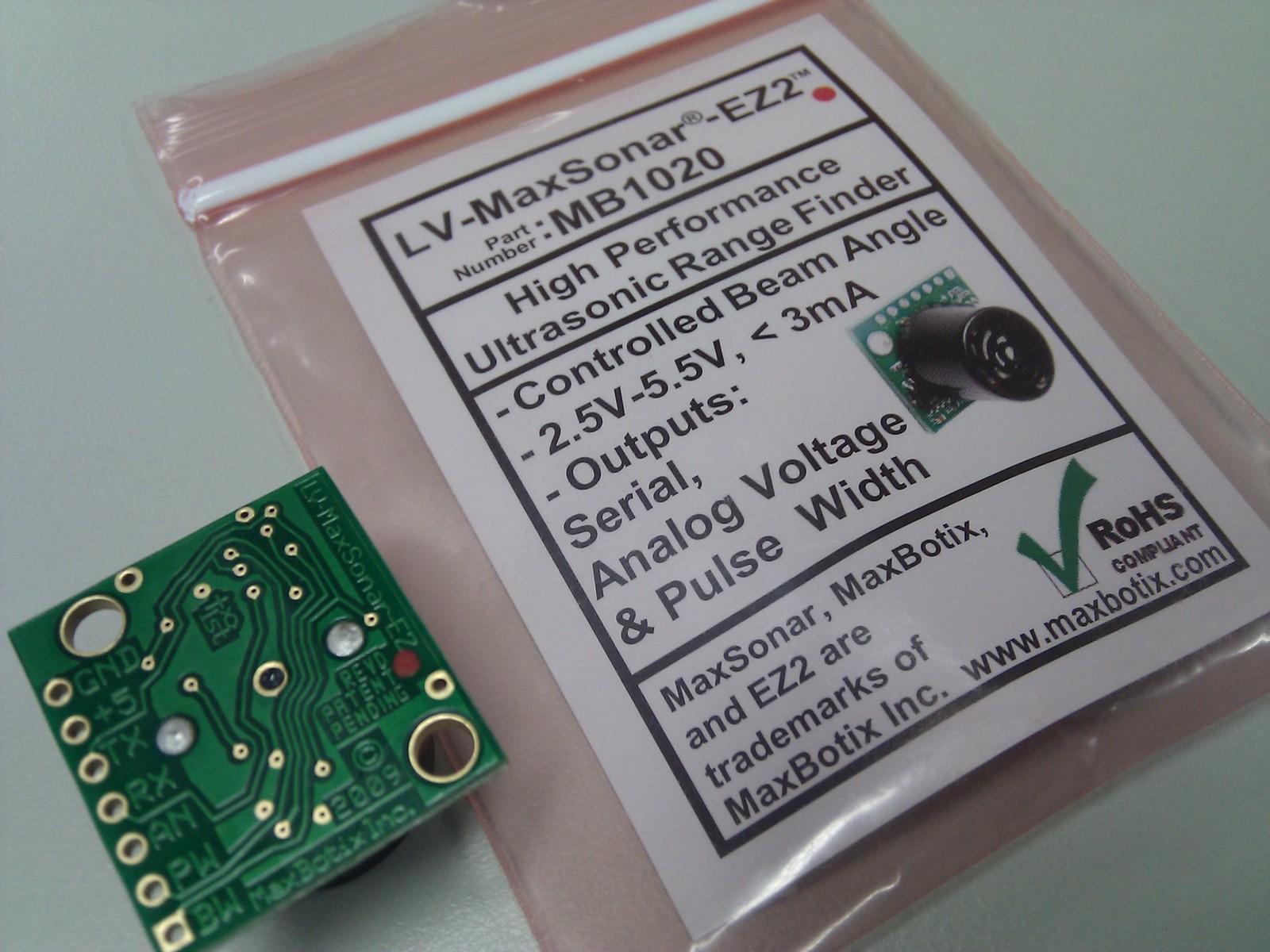This detailed photograph captures a green computer chip adorned with embedded transistors and small gold circles connected by intricate green lines. Adjacent to this chip is a pinkish-translucent Ziploc bag featuring a white label with black text. The text on the label reads: "LV-MAX SONAR EZ-2. Part number MV1020. High performance ultrasonic range finder. Controlled beam angle, 2.5V to 5.5V, less than 3MA. Output: serial analog voltage and pulse width." The label also states that "MAX SONAR," "MAX BOTIX," and "EZ-2" are trademarks of MAX BOTIX, Inc., and includes the website "maxbotix.com" with a green checkmark above it. A black cylinder appears to be part of the equipment, and there's an illustration of a fan or similar component on the chip, implying its function or structure. The packaging background has a brown tint, enhancing the contrast with the white label and the green circuit board.